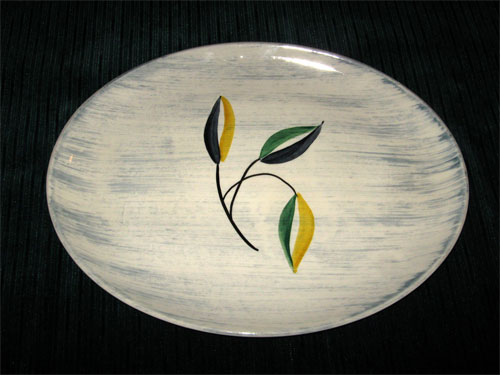The photograph features an oval-shaped plate captured from above at a slightly oblique angle, giving it an elongated appearance. The plate, which appears to be made of shiny glass or ceramic, has an off-white or cream background adorned with delicate blue horizontal stripes that intensify in color toward the edges. Centered on the plate is a stylized illustration of three stems, each bearing leaves in various hues of green, white, black, and gold. The left stem curves inward and sports a green leaf, while the right stem holds a gold leaf. The third stem, pointing downwards, mirrors the left stem with its green hue. The plate is set against a stark, featureless black background that accentuates its glossy surface and detailed design. The overall style of the image is realistic, capturing the intricate details and textures of the plate with a high degree of photographic clarity.